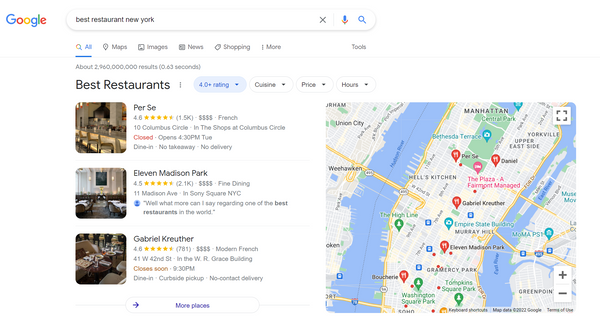The image depicts a Google search results page with the query "best restaurant in New York" entered in the search bar. The search bar, located at the top center of the page, features the Google logo on the far left, followed by the user input, and to the right, icons for clearing the search (X), voice search (microphone), and search (magnifying glass). Below the search bar, navigation options such as All, Maps, Images, News, Shopping, More, and Tools are visible, with 'All' being highlighted.

The page indicates that there are approximately 2,960,000 results for the search query. Directly below this information, a highlighted filter option labeled "Best Restaurants" is visible. To the right of it, there are filtering options including "4.0 rating plus," which is highlighted, alongside "Cuisine," "Price," and other selection icons.

Beneath these filters, a list of three highly-rated restaurants is shown: Per Se, Eleven Madison Park, and Gabriel Kreuther. Each restaurant has over 4.5 stars, with Eleven Madison Park having the lowest rating among them at 4.5 stars. All three establishments are marked with four-dollar signs ($$$$), indicating a high price range.

At the bottom of this section, there is a prompt to view more places.